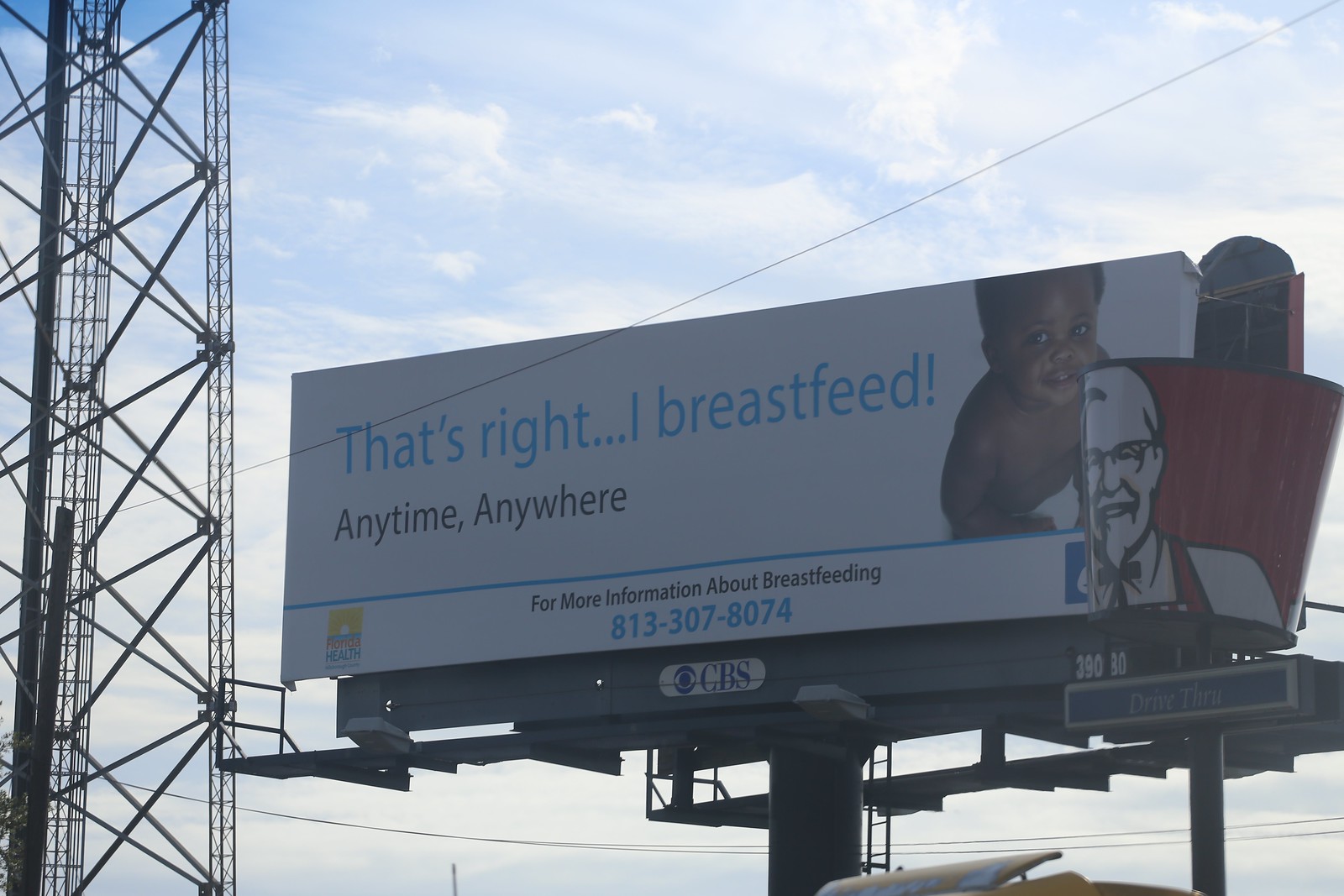The image captures a large, rectangular billboard mounted on a tall metal post, typically found alongside a highway. The billboard features a plain white background with bold blue text at the top reading, "That's right… I breastfeed!" followed below in smaller black letters with "Anytime, anywhere." In the upper right-hand corner, there's a photograph of an African-American baby boy wearing a diaper, sitting and looking up with a smile. At the bottom of the billboard, it provides a phone number for more information about breastfeeding. To the right of the billboard, there is a sign for a Kentucky Fried Chicken restaurant, prominently displaying the iconic bucket with Colonel Sanders' face. On the left, tall electrical towers and power lines stretch across the sky, framing the billboard. The scene captures a blend of commercial advertising and essential public health messaging.